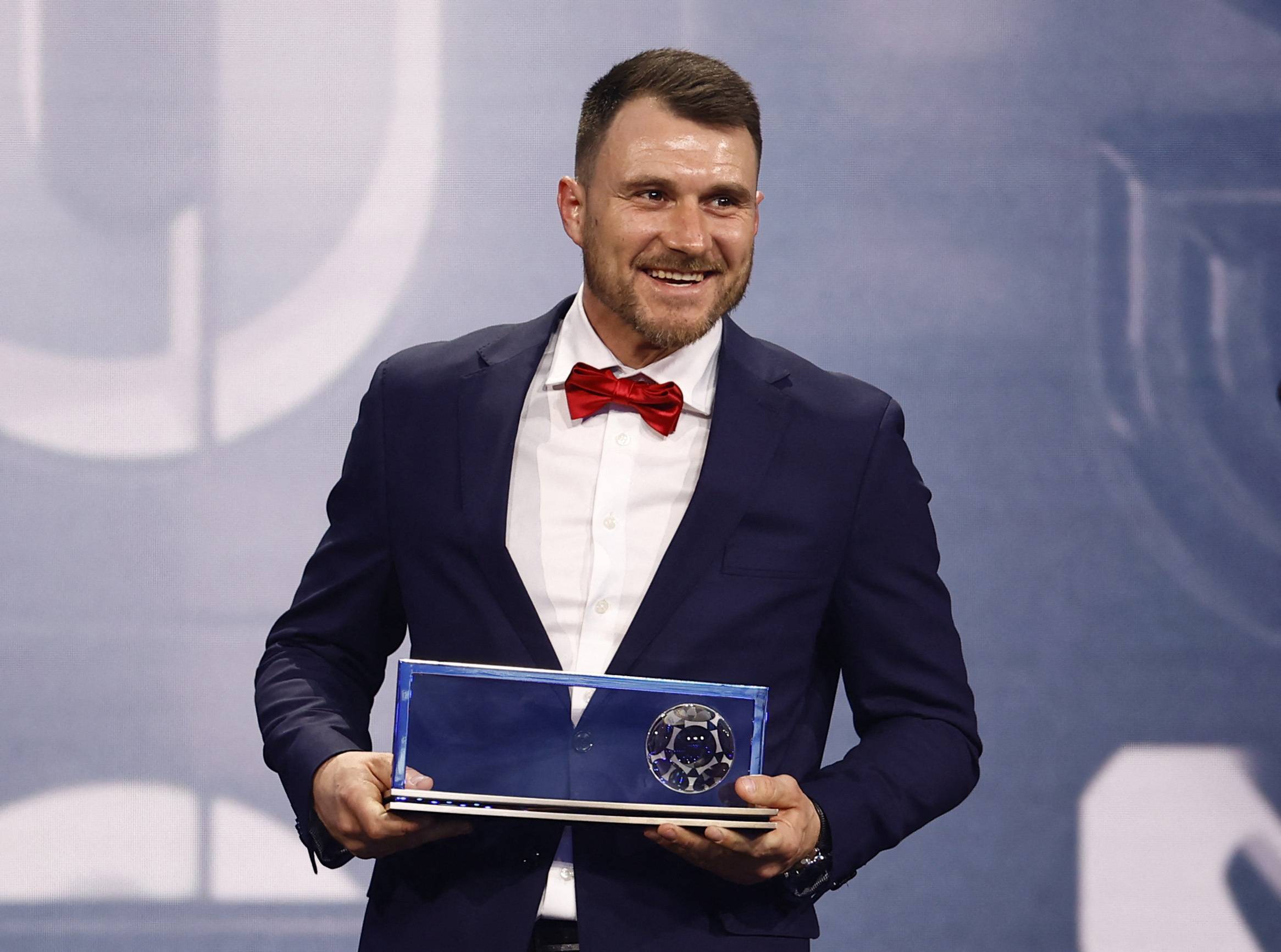In this landscape-oriented photograph, the main focus is a Caucasian man standing proudly and possibly receiving an award. He is dressed in a modern navy blue suit jacket, a white dress shirt, and a striking red bow tie. The man, who has short brown hair and a well-groomed beard, is looking slightly to his left with a big grin on his face. He holds an award that features a metal base with a horizontally oriented glass or plexiglass slab tinted blue, through which the button on his sports coat is visible. On the right-hand side of this slab, there is an image resembling a soccer ball. The backdrop behind him is composed of varying shades of blue with some lighter areas, featuring logos or words that are too large to be fully legible. This backdrop, however, accentuates the formal and celebratory nature of the scene.